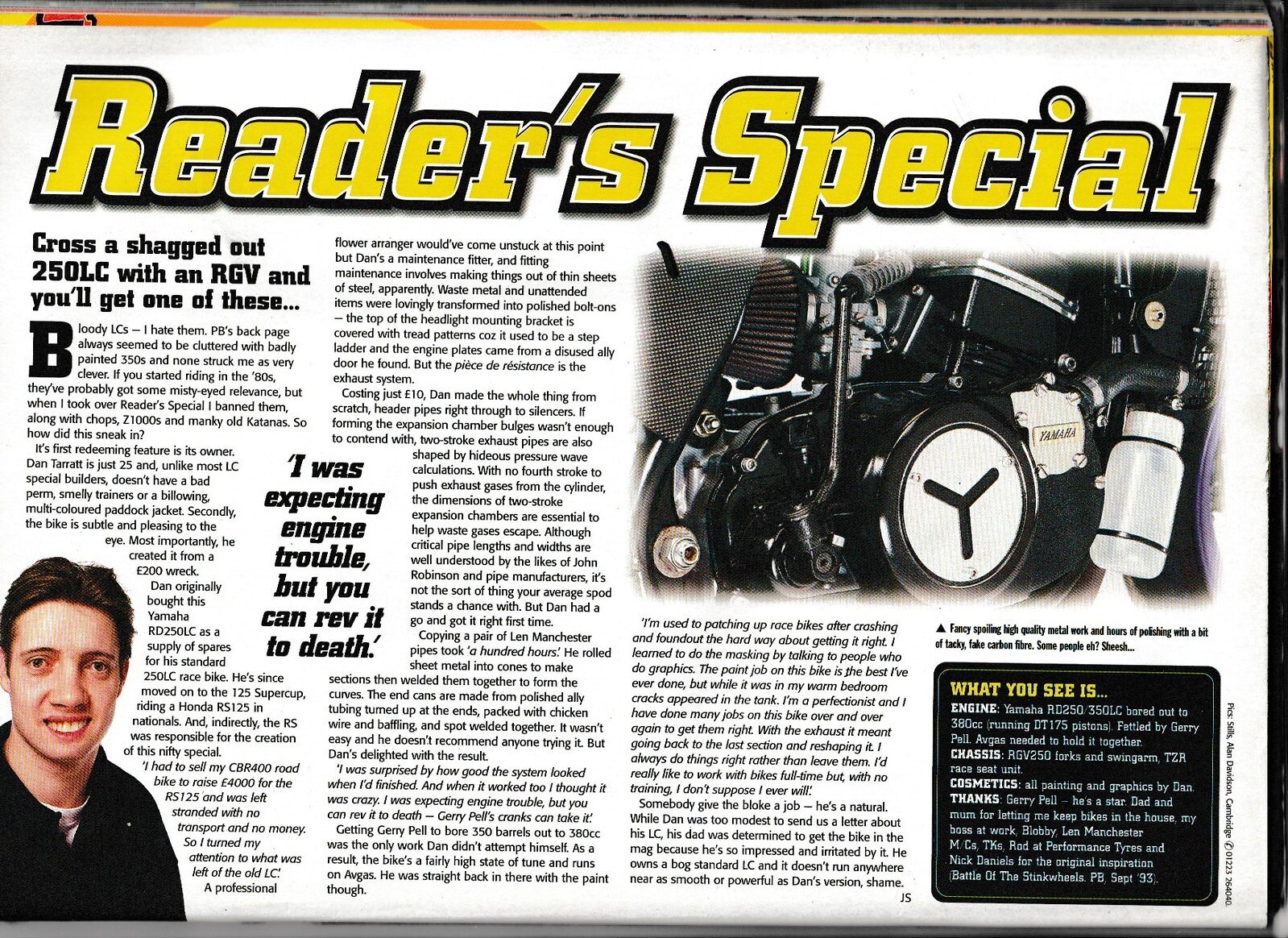This detailed snippet from an automotive magazine features an article titled "Reader's Special" prominently displayed in bold yellow letters against a white background. The article, written in black font, is centered around the intriguing headline: "Cross a shagged out 250 LC with an RGV and you'll get one of these." The layout includes a detailed discussion about engines, especially highlighting a Yamaha motorcycle engine. At the bottom left of the article, there's a picture of a young man wearing a black sweatshirt, his dark hair complementing his cheerful expression. Adjacent to his photograph, towards the top-right corner, there’s an image showcasing the intricate details of a motorcycle engine. Additionally, the article provides a brief synopsis focusing on engine specifications, chassis details, and other terminologies relevant to car and motorcycle enthusiasts. It concludes by acknowledging contributors, emphasizing its informative and engaging content for those passionate about automotive engineering.